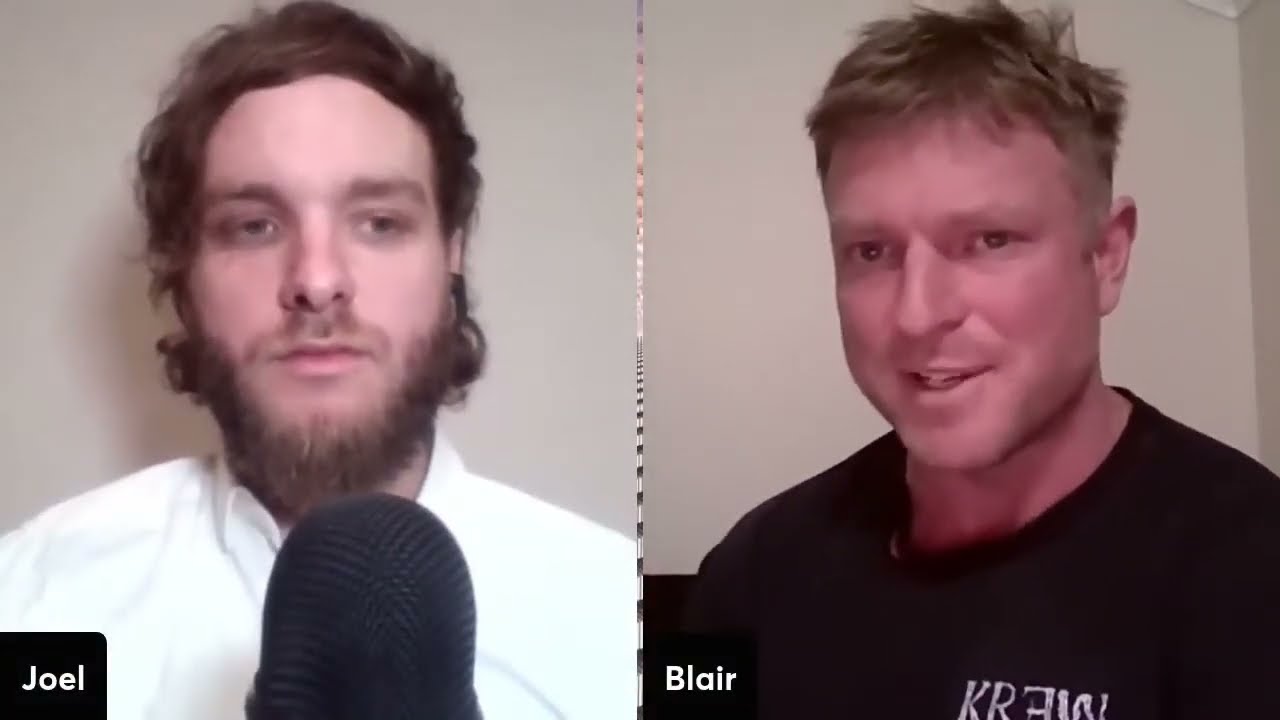The image features two juxtaposed photos of men against beige or tan walls. On the left side, Joel is standing in front of a beige wall. He has brown, curly hair, a full brown beard, and a light mustache. He is wearing a white collared shirt and speaking into a prominent gray microphone. His name, "Joel," is displayed in a black box with white font at the bottom left corner of his photo. On the right side, Blair stands against a similarly colored wall with short blond hair and noticeably reddish skin. He is wearing a black t-shirt that has "K-R-E-W" printed on it, with the 'E' reversed. Blair is looking slightly to the left and has his name displayed in the same style black box with white font at the bottom left corner of his photo. The image as a whole exhibits both men’s contrasting appearances and environments.